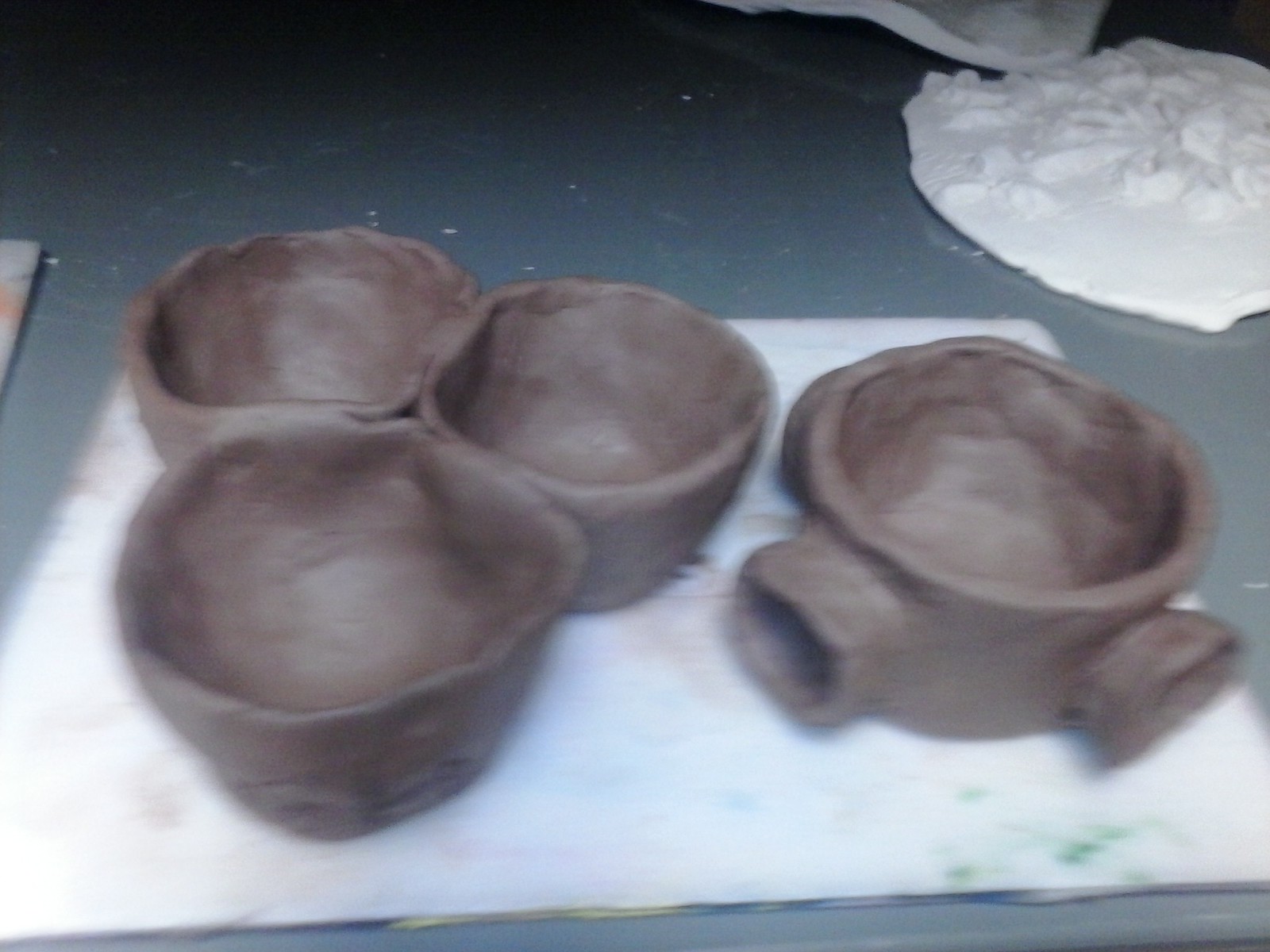This detailed color photograph captures an assortment of brown clay pottery pieces, in the midst of being crafted. Three roughly formed, uneven cups are positioned on the left, while a fourth piece, resembling a kettle or a spouted pot, is on the right. These ceramics rest on a white, smudged surface that appears marked with various clay stains and other colors. The entire setup is on a slab of slate-gray material, with white flecks throughout. The background features a white board adorned with what looks like a decorative, dried piece of ceramic or porcelain, exhibiting a faint floral design. A stained cloth, mottled with brown and green hues, adds to the rustic, artisan ambiance of the scene.